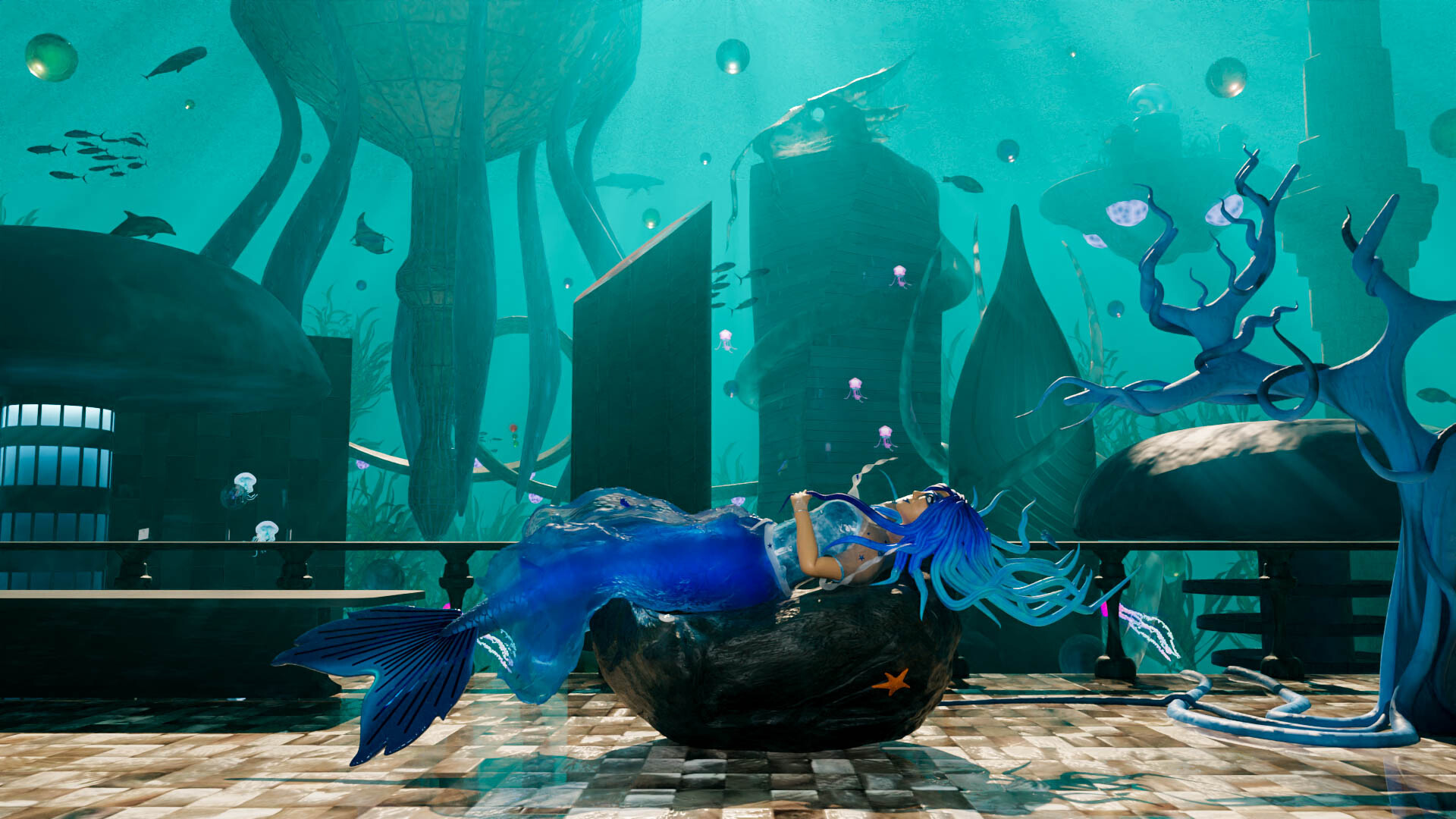The image depicts a highly detailed, computer-generated scene that exudes a nostalgic, early 2000s aesthetic, reminiscent of old-school graphic rendering. It portrays an underwater fantasy setting, possibly inspired by a music video or a scene from a video game. Central to the image is a mermaid with distinctive, spiked blue hair that resembles Medusa's snake-like locks or squid tentacles. She rests languidly on a large shell or pillow amidst a futuristic city submerged in the depths of the sea. Surrounding her are an assortment of marine life, including fish, dolphins, and possibly stingrays, swimming among the strange, otherworldly structures and aquatic vegetation that make up this vivid, mythical underwater world.